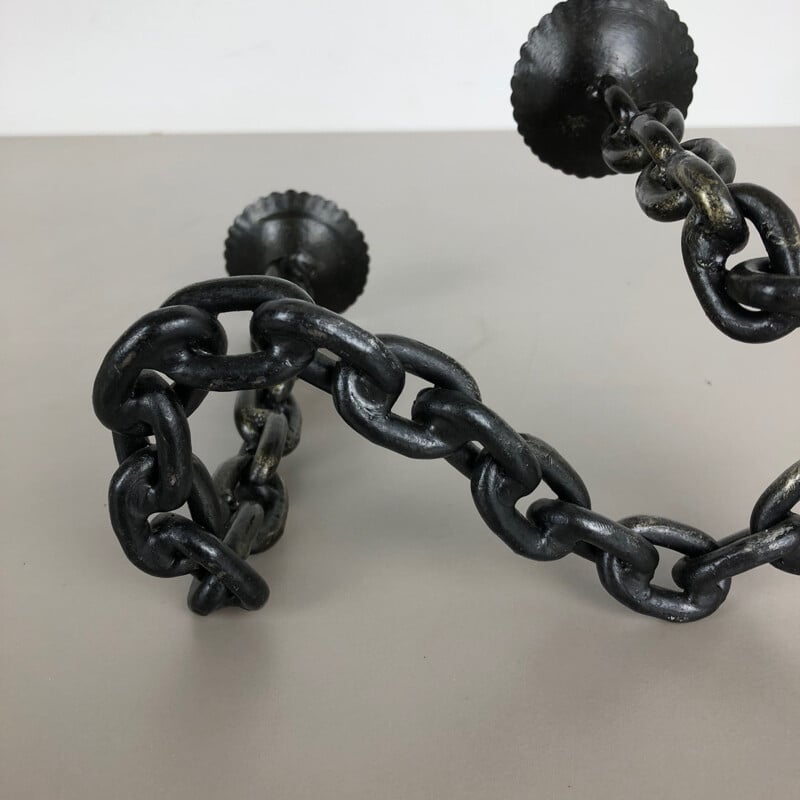The image depicts a detailed scene featuring a black iron chain arranged in an intricate pattern on a grayish-white surface, possibly a table or floor, against a pure white wall backdrop. The chain, made of thick metal, forms a zigzag layout and includes several scalloped, seashell-like metal plates or caps at both visible ends. One portion of the chain appears to rise vertically before bending horizontally and then diagonally descending, illustrating a complex and seemingly gravity-defying arrangement. The chain's sections shift between lying flat, descending, and reascending, adding to the curiosity of how it maintains its form. The combination of the iron chain's dark coloration and the light surface beneath accentuates its contours and details, presenting a visually striking composition that could be interpreted as a piece of artwork.